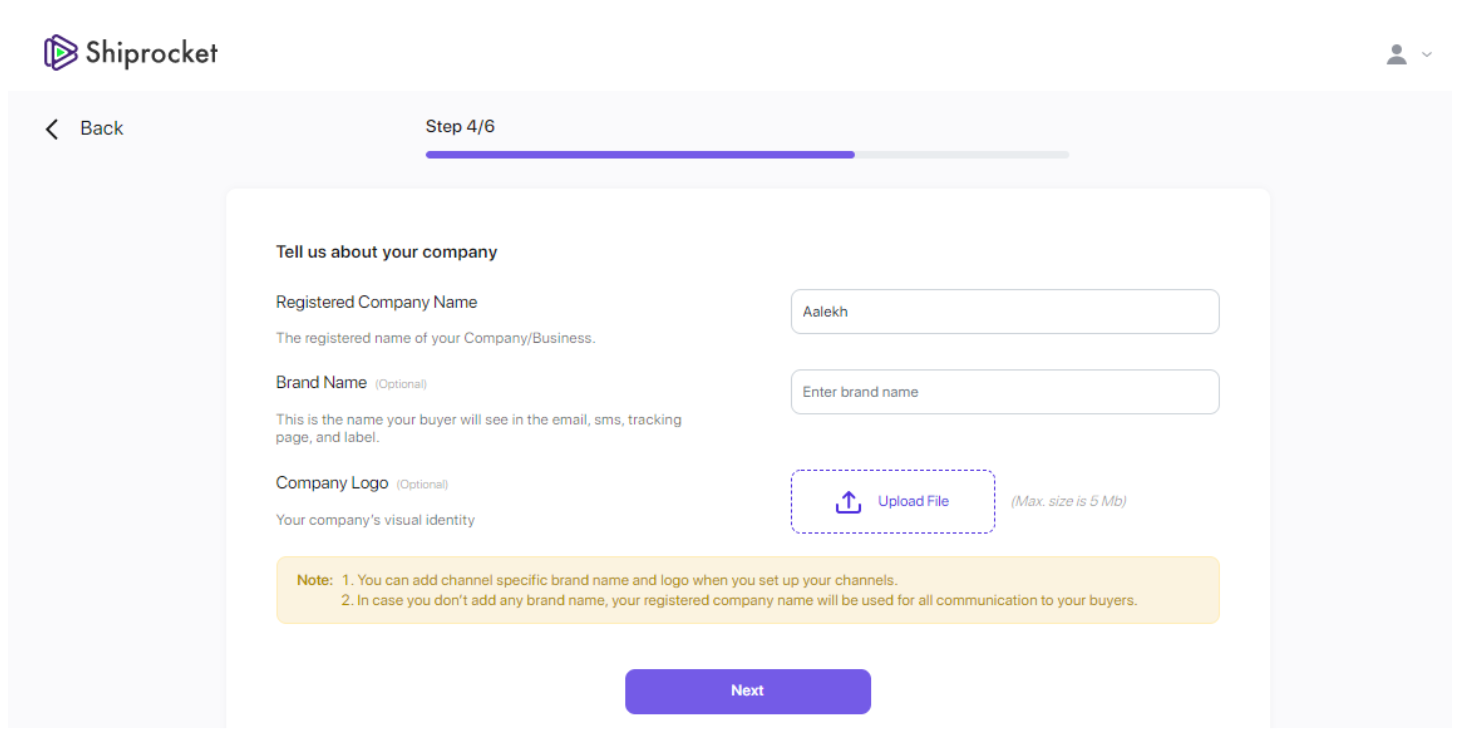The image is a screenshot from a webpage with a white background, presenting a section of the Shiprocket software interface. In the upper left corner, the company name "Shiprocket" is displayed in a dark gray font, with a capital 'S' followed by lowercase letters. Adjacent to the name is the company logo, which consists of two superimposed triangles with a small aquamarine green speck in the middle.

At the center of the image, the text "Step 4 of 6" is prominently displayed, indicating the current stage in the configuration process. Below this step indicator, the heading "Tell us about your company" appears. The first field requests the "Registered Company Name," adjacent to which is a text input box where the name "alekh" is filled in.

The next field, labeled "Brand Name (Optional)," informs users that this is the name buyers will see in emails, the tracking page, and labels. Below that, there is a section for the "Company Logo (Optional)," accompanied by an upload box. This box features a purple "Upload File" button with an upward-pointing arrow.

Further down, a light pink rectangle with brown font provides additional notes. 1) Users can add channel-specific brand names and logos when setting up their channels. 2) If no brand name is added, the registered company name will be used for all buyer communications.

Finally, a purple rectangle at the bottom with the word "Next" in white signifies the progression button for moving to the subsequent configuration step.